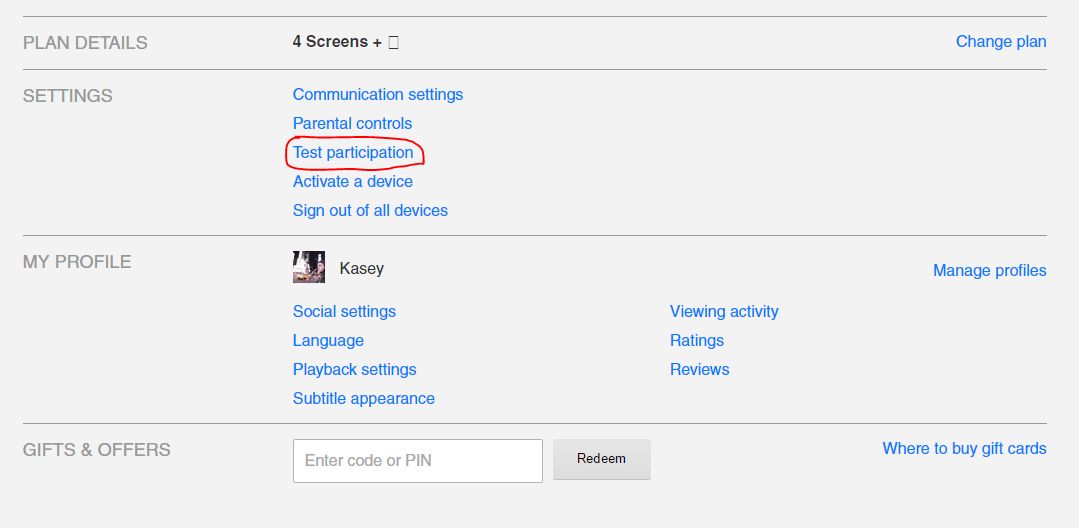The image depicts a website interface resembling popular streaming services such as Netflix or Hulu. The layout suggests a user account control panel with various options and settings. Highlighted features include the ability to watch content on four screens and the option to change the subscription plan, the latter highlighted in blue. 

The interface presents several tabs, including "Settings," "My Profile," and "Give Offers." Under "Settings," options such as "Communication Settings," "Parental Controls," "Test Participation," "Activate a Device," and "Sign Out All Devices" are listed, with "Test Participation" notably circled in red.

In the "My Profile" section, the user Casey is noted along with a small, unclear profile picture. Sub-options under this section include "Social Settings," "Language," "Playback Settings," "Subtitle Appearance," "Viewing Activity," "Ratings," "Reviews," and "Manage Profiles," all highlighted in blue.

The "Give Offers" section allows users to enter a code or pin to redeem offers and provides information on where to purchase gift cards. The background has a grayish-white hue, accentuating the control panel elements, suggesting this is indeed a movie or streaming website's settings page.